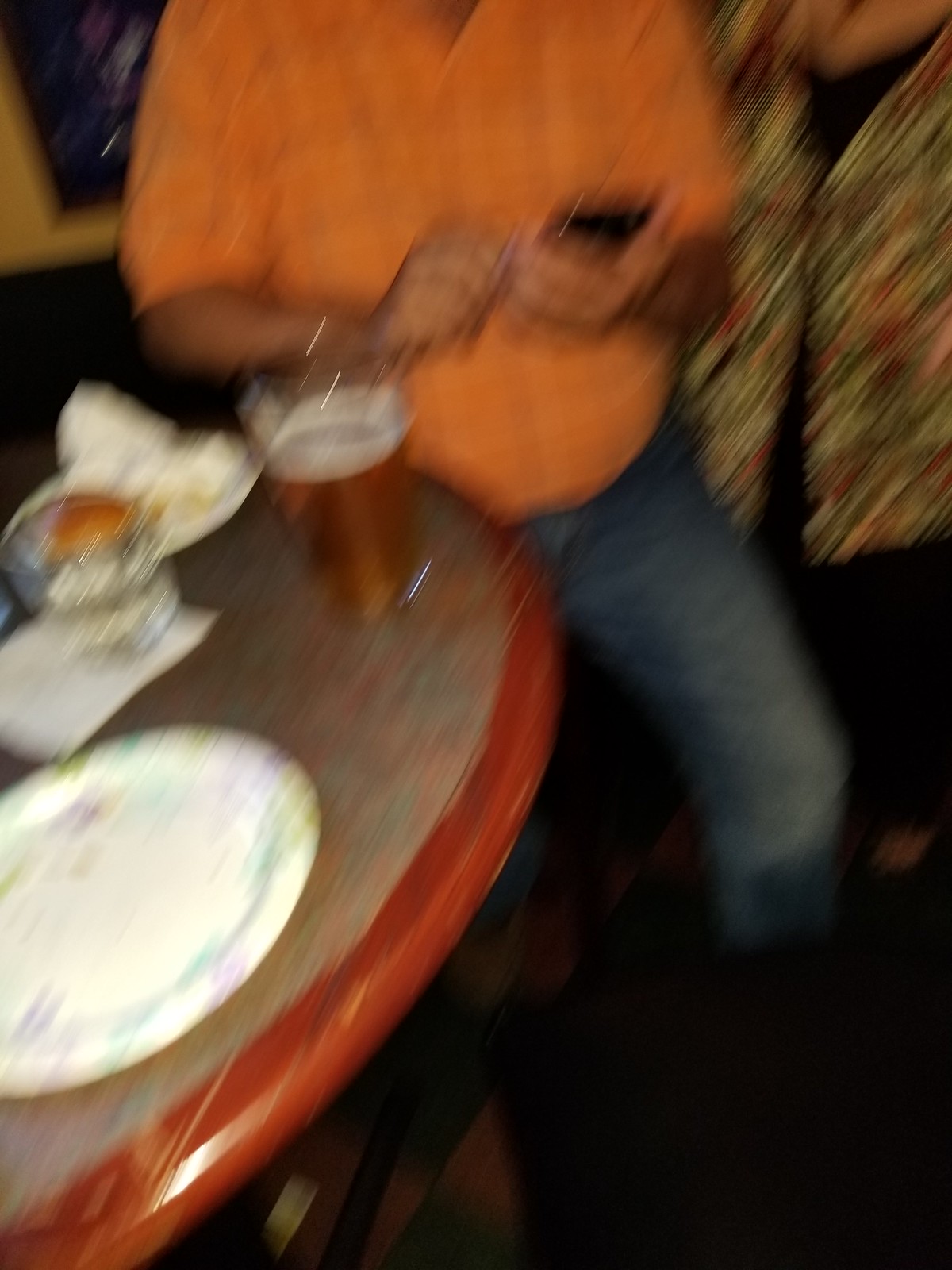In this slightly blurry photograph taken at a restaurant, the left side features about half of a round table. On this table, there is an empty plate and another plate with what appears to be the remnants of a hamburger wrapped in foil. Scattered across the table are a few napkins and a mostly full cup of beer, approximately three-quarters full. In the background, there seems to be either a window or a picture on the wall.

To the right side of the image, the torso of a man dressed in a button-down orange shirt and jeans is visible. He is holding a phone in his left hand, seemingly engaged with it. Adjacent to him, on the left side of the image, stands a woman dressed in a black and gold jacket over a white shirt, paired with black pants. Her head is also not visible in the frame. The partially obscured figures and the casual disarray on the table hint at a relaxed dining atmosphere.